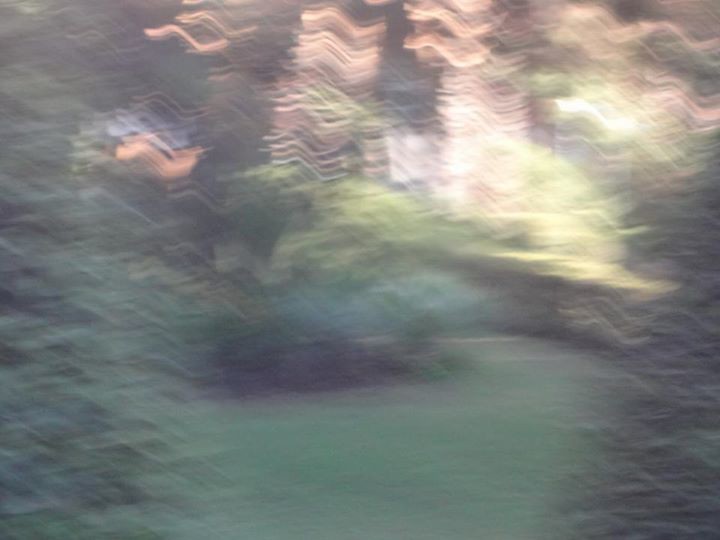This image is an abstract, rectangular photograph, oriented horizontally with its long side from left to right. The overall scene is very blurry with no immediately discernible objects, suggesting motion blur or digital alteration. The bottom of the image is dominated by solid green, resembling grass, with potential shrub-like shapes indicated by shadows. Flanking this, on both the left and right, the green areas continue but maintain the same indistinct quality. As the eye moves upwards from the green base, the colors transition into lighter shades including yellows, golds, and oranges. These lighter colors form horizontal squiggly lines, zigzagging akin to elongated, angular S-shapes. These colors create an impression of dynamic movement, with some people describing the shapes as sharp, triangular, or stacked in a three-point pattern. In the midst of this blurred landscape, near the center, vague human-like features can be inferred—possibly a light green top and darker green lower half, and what might be interpreted as an eye and eyebrow—but these are unclear and may simply be the result of the abstract nature of the image.